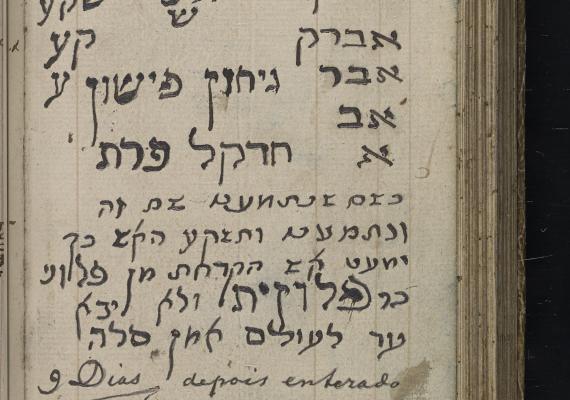The image depicts a very old, thick book with what appears to be equally thick, ruffled pages. The book is open, showcasing a page dominated by lines of text that are not in English. The upper half of the page features hieroglyphics or possibly Hebrew script, given the intricate and varied handwritten letters, which are dark gray in color against the off-white, lightly marked background. The text is right-justified and intricately detailed. At the bottom of the page, there are several words in cursive, such as “Dias,” “Dipois,” and “Enterado.” The entire book seems to be framed, with a visible light brown to beige border, taking up most of the image except for a black stripe on the right side, indicating a dark background. The overall orientation of the image is slightly wider than it is tall, giving it a subtle landscape appearance. The frame edges are visible on the right side and barely on the left, while the top and bottom edges are not within the image's scope.